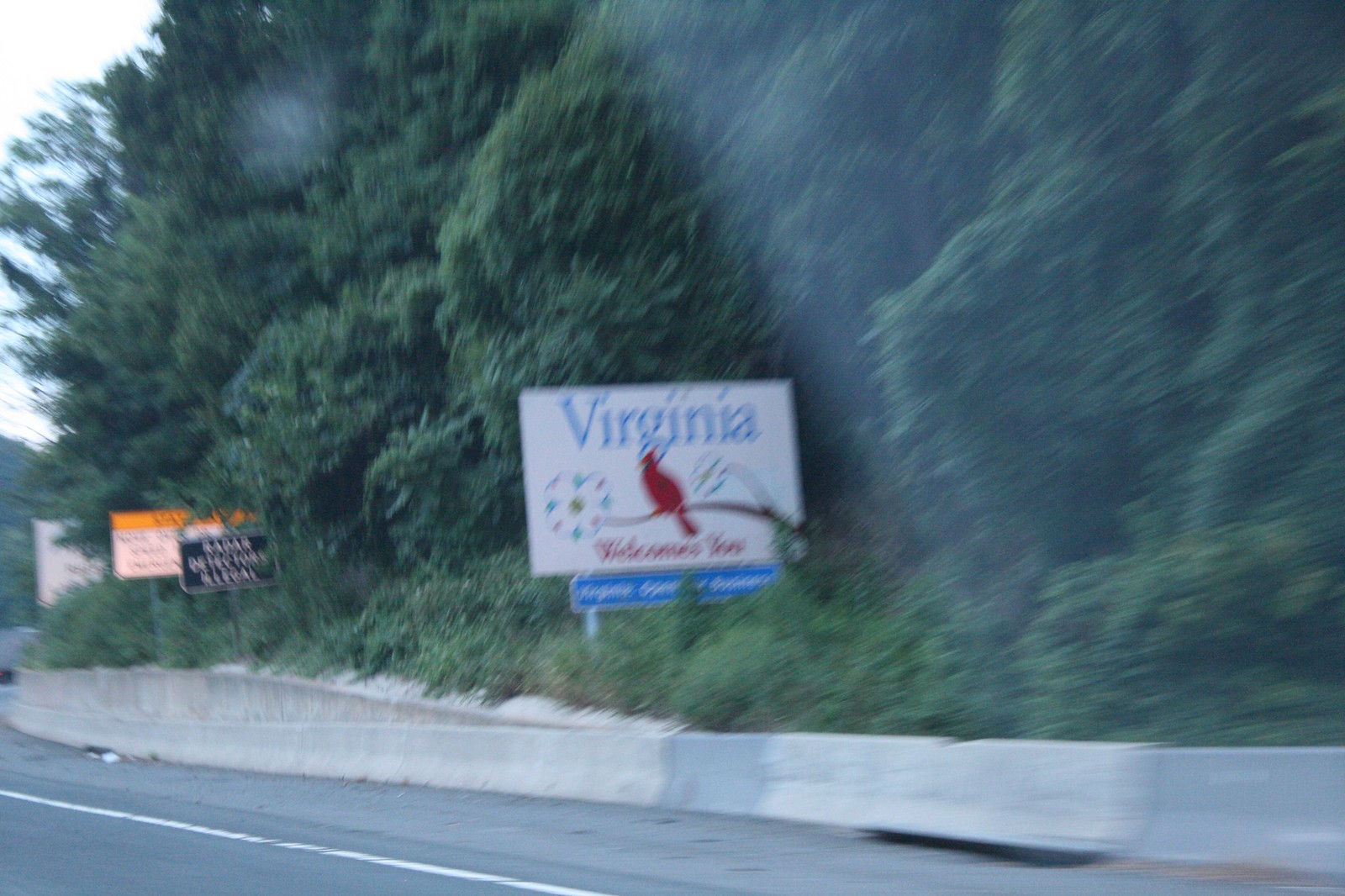This somewhat blurry photograph captures the bustling atmosphere of a highway scene with several detailed elements. The dark gray, nearly black concrete surface of the road is discernible along with a distinctly visible white line marking. An imposing concrete retaining wall flanks the highway, partially covered by thick, healthy green shrubbery that includes dense bushes and towering trees. Prominently featured is a distinctly visible white sign with blue font, indicating the state of Virginia. Perched on a branch underneath the text is a vibrant cardinal, adding a splash of red to the scene. Below the bird, in red font, the words "welcomes you" are clearly visible. Additionally, a secondary blue sign with white font is situated below the welcoming message. Multiple road signs are present, including a black one with white font, a white one with a gold strip at the top, and another white sign partially obscured behind them. The image is slightly obscured by lens flare, adding a touch of artistic imperfection to the otherwise detailed snapshot.